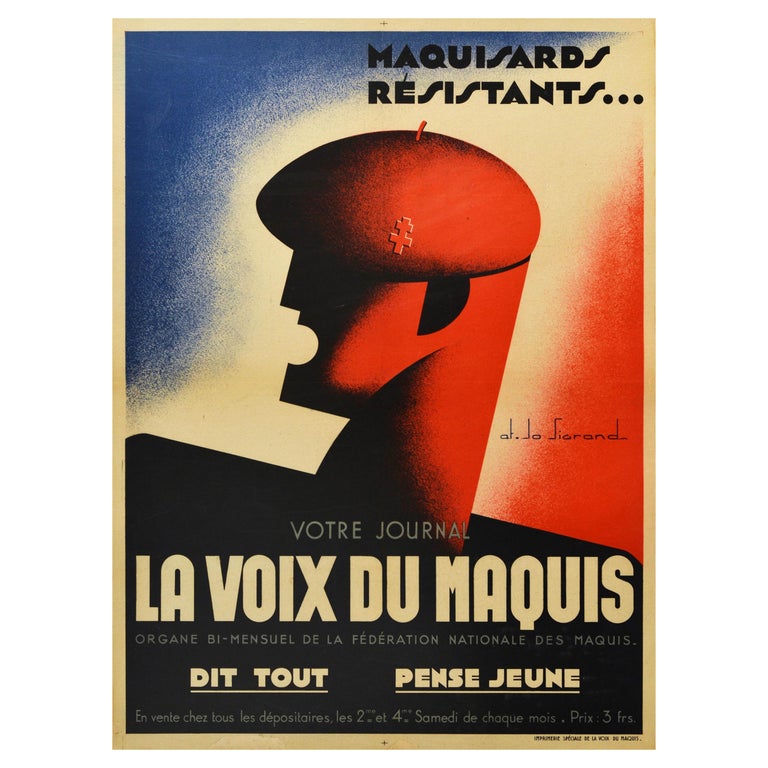The image is of a detailed French-language poster with a tricolor background of blue, white, and red from left to right. It features a caricature drawing of a man, predominantly colored in red, with his lower frame gradating to black. The man is wearing a red beret adorned with a puzzle piece above his right ear. His mouth is open as if he is speaking or yelling, and his features are stylized to look like interconnected puzzle pieces, deviating from a normal human illustration. The poster has a thin white border and black text in the lower right corner. Prominently at the top right, the text reads "MAQUISARDS" followed by "RESISTANTS" with three periods. Below the caricature, the words "VOTRE Journal," "La Voix du Marquis," and smaller text stating "Organe par Mansuel de la Fédération Nationale du Marquis d’Itout-Pens-Jouan" and the artist's signature "Dito Fernando" are present.